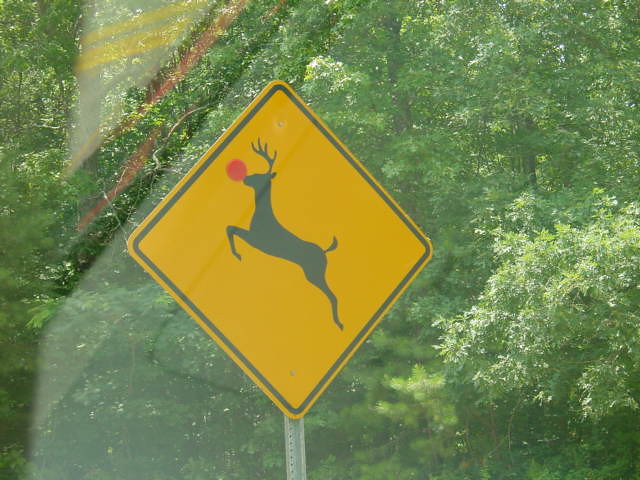This photograph, taken outdoors through the window of a vehicle, captures a deer crossing sign situated on a silver metal post. The sign is a yellow diamond with a black border and features a silhouette of a deer in mid-jump, adorned with a conspicuous red dot on its nose. The background reveals a mix of trees and shrubbery, with sunlight filtering through the foliage, casting an ethereal glow. The overall image has a reflective sheen, indicative of the photo being shot through a windshield. The detailed scene merges natural and man-made elements, with the forested area providing a serene contrast to the alertness of the deer crossing sign.